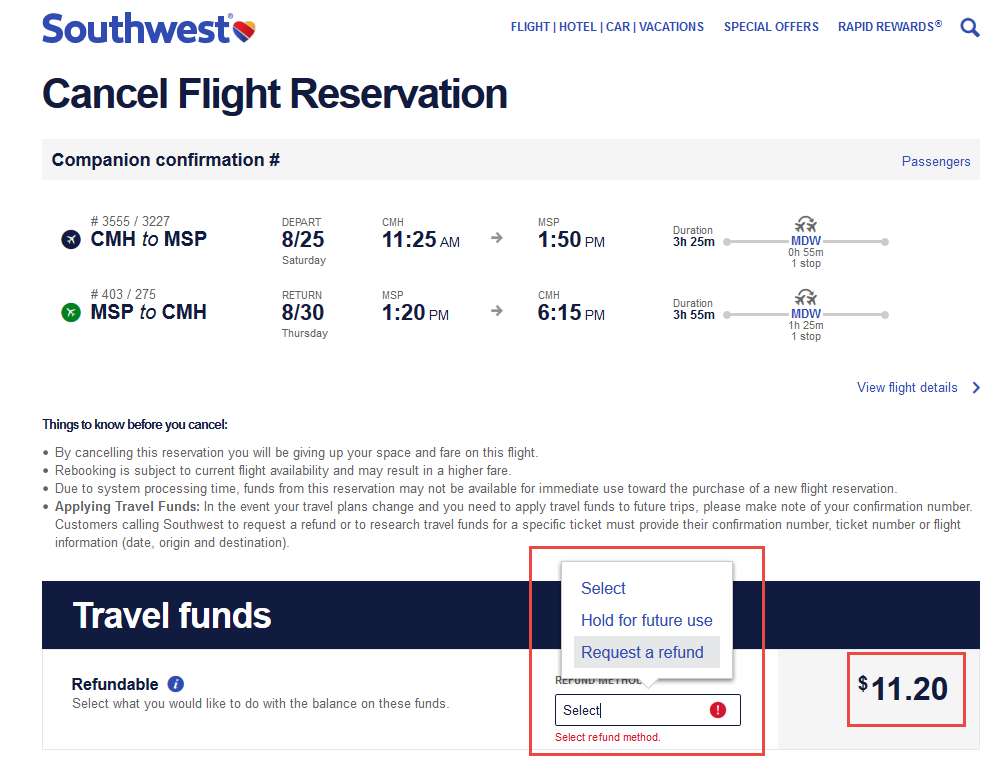This detailed screenshot from the Southwest Airlines website displays the Gansol flight reservation section. In the upper left corner, the heading reads "Southwest Gansol Flight Reservation." Centrally located towards the right are menu options including Flight, Hotel, Car, Vacation, Special Offers, Rapid Rewards, along with a search icon.

On the left-hand side, detailed itinerary information is provided. The companion's confirmation number shows a flight from Columbus (CMH) to Minneapolis-St. Paul (MSP) departing on Saturday, August 25th at 11:25 AM and arriving at 1:50 PM, with a total duration of 3 hours and 25 minutes, including a stop at Chicago Midway (MDW). The return flight from MSP to CMH is scheduled for August 30th at 1:20 PM, arriving at 6:15 PM, totaling a duration of 3 hours and 55 minutes, with a 1 hour and 25-minute layover at MDW.

Additional details include a link to view the full flight details and an advisory note stating that canceling the reservation will forfeit the reserved space and fare on the flight. Rebooking the flight is dependent on current availability and may incur higher rates.